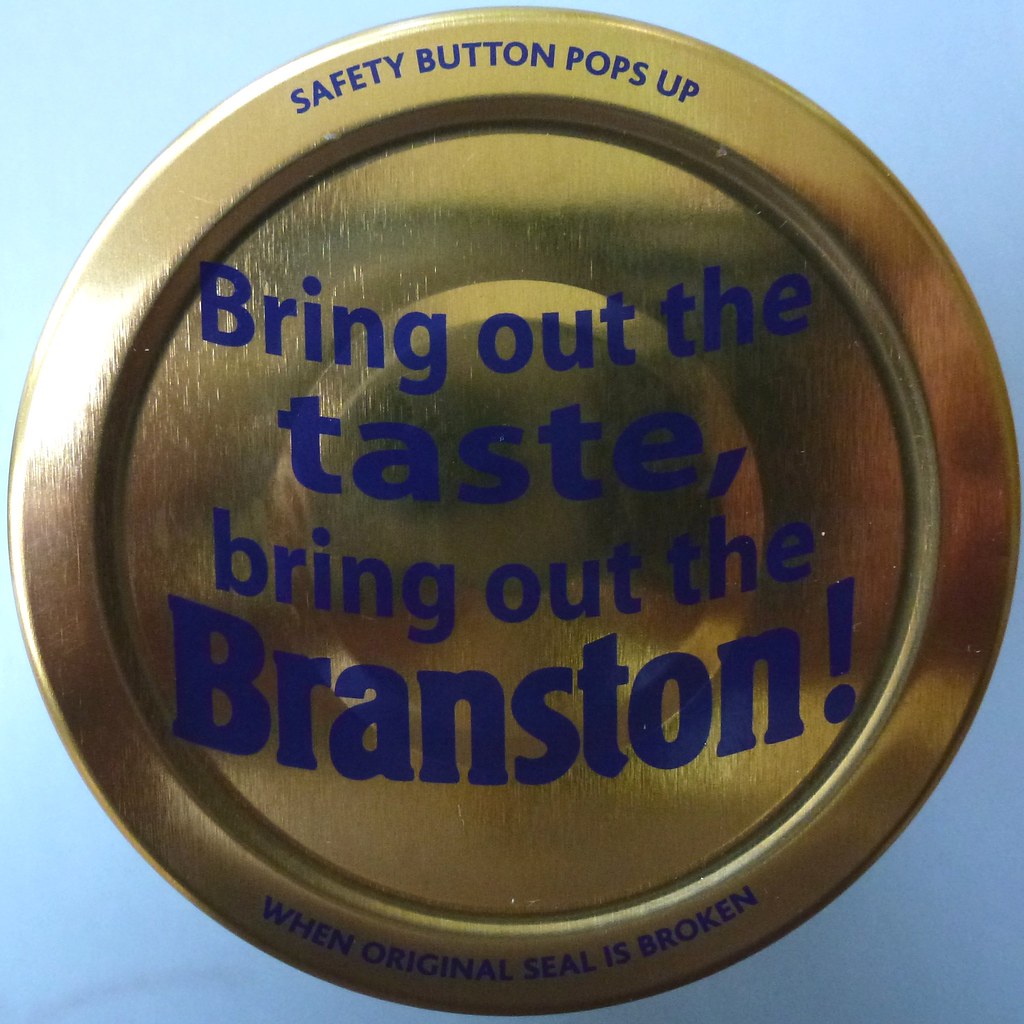This photograph captures a close-up of a golden tin lid that prominently features embossed sides and faint scratches. The lid is vertically positioned, facing the camera, and rests against a background that transitions from a bluish-white gradient, darker on the right side, to a lighter tone on the left where a light source reflects off its surface. Encircling the rim of the lid, in uniform blue font, the text reads "Safety button pops up when original seal is broken." Centrally placed, in larger blue letters, is the slogan "Bring out the taste, Bring out the Branston," with "Branston" being the most prominently featured word. Notably, the safety button on the lid has been activated, indicating the seal has been broken.